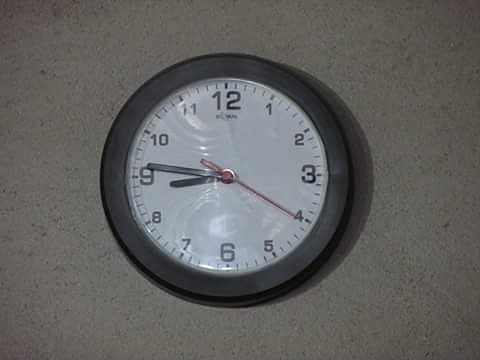The photograph depicts a plain, businesslike wall clock mounted on what appears to be a textured, tan wall that has the appearance of aged stucco. The clock itself features a thick black frame that seems slightly worn and scuffed, indicative of heavy use. Centered in the image, the clock has a stark white face with black numerals from 1 to 12, with the 12, 3, 6, and 9 appearing in a larger print. The hour and minute hands are black, as is the second hand, which is currently pointing at 20 seconds. The time displayed is 8:46. There is noticeable reflection on the clock’s glass covering, adding to the slightly fuzzy and worn feel of the entire image.